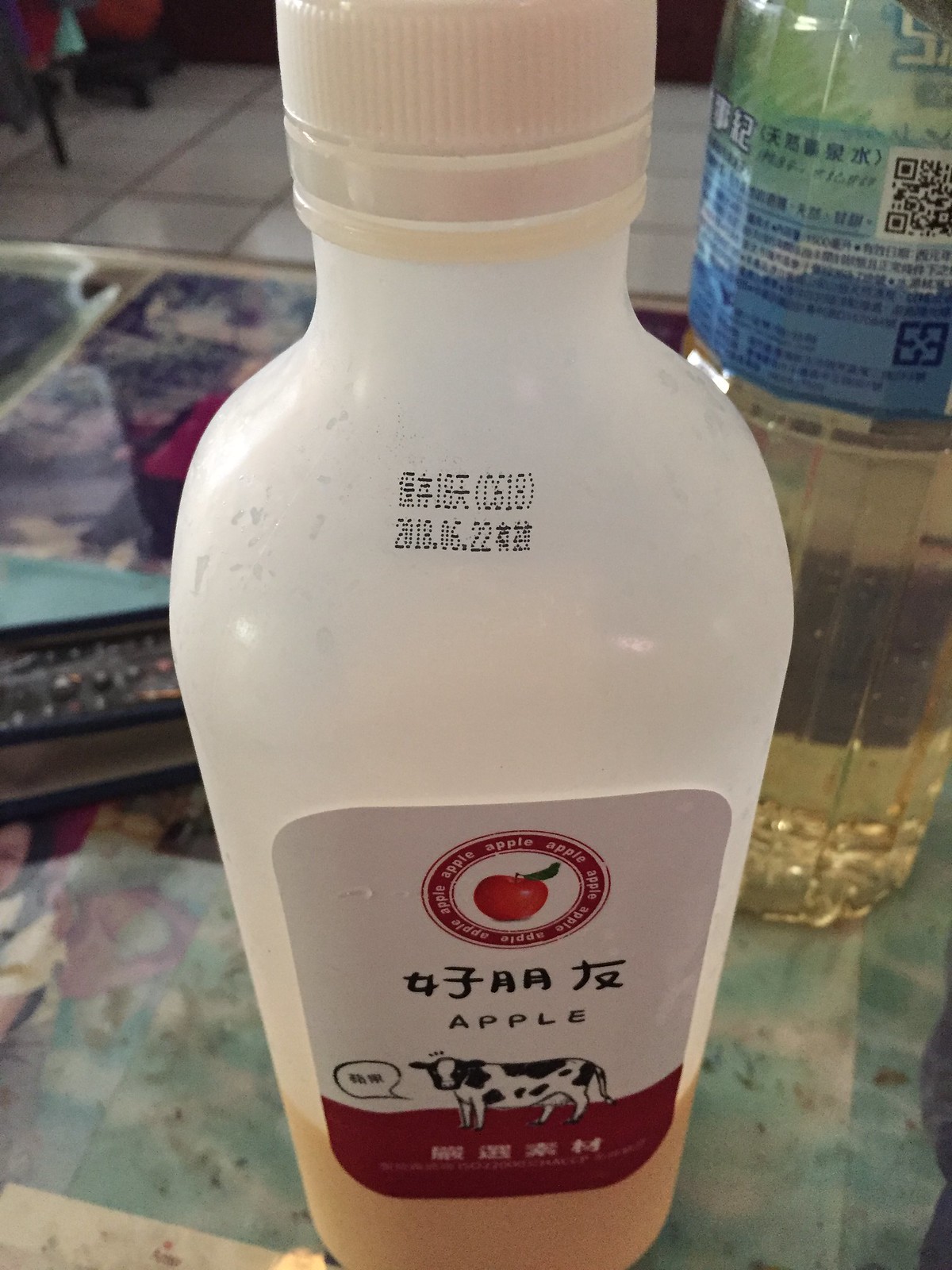This photograph captures an extreme close-up of a glass tabletop, likely situated in a kitchen or diner, with a white tile floor visible in the background. On the table is a colorful placemat. Foremost in the image are two bottles with labels featuring Asian script. The bottle closest to the camera is a clear plastic bottle with a white screw cap, containing beige-colored apple juice and labeled with an illustration of an apple flanked by a red circle and green leaf, followed by the word "apple" and more Japanese text. Additionally, a black and white cow is depicted on the label, looking directly at the viewer with a speech bubble inscribed in Japanese. This bottle is about a quarter full, indicating it has been partially consumed. The second bottle, positioned to the right and partially cut off by the edge of the image, displays a blue and green label with a QR code and Asian text, and contains a yellowish liquid that might be tea. The background reveals reflective white square tiles, enhancing the brightly lit and clean appearance of the scene.